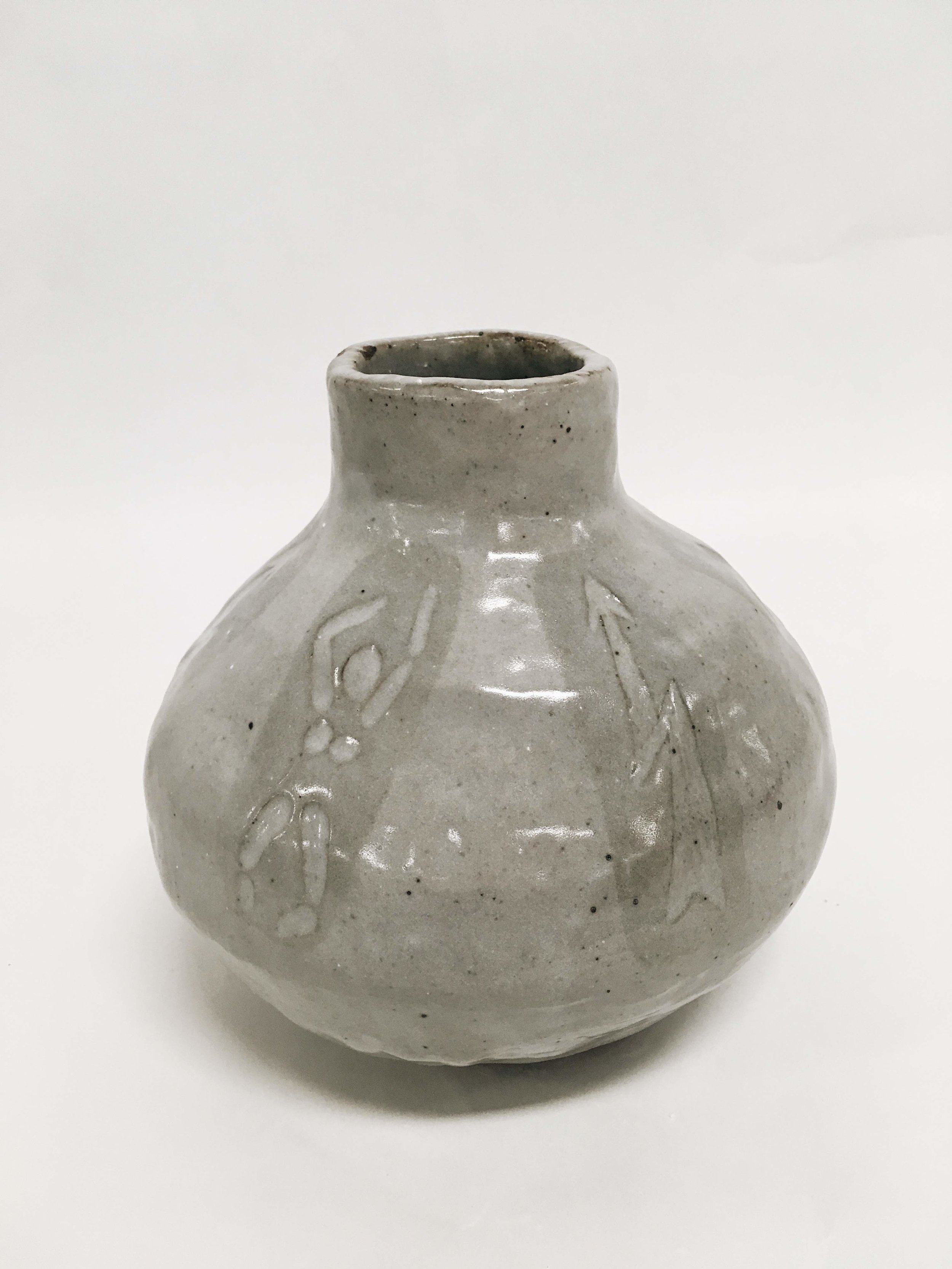The image depicts a short, stubby, and round ceramic vase with a glossy, shiny finish. The vase features a grayscale color palette, dominated by varying shades of gray and dark gray, adorned with thinly scattered black speckles. The design on the vase includes a vertical figure resembling a person with arms raised overhead, distinctly visible on the left. Adjacent to this figure, to the right, is an arrow pointing upwards, possibly with another object or arrow beneath it. The vase's body tapers into a pipe-like shape near the top, culminating in an open hole, suitable for holding plants or other items. The entire scene is set against a pure white background, possibly achieved using a piece of paper for a cleaner photographic presentation, highlighting the vase as the central object in a minimalist composition. The vase's design mixes abstract human forms with simple geometric elements, making it suitable for home decor or display in a modern setting.